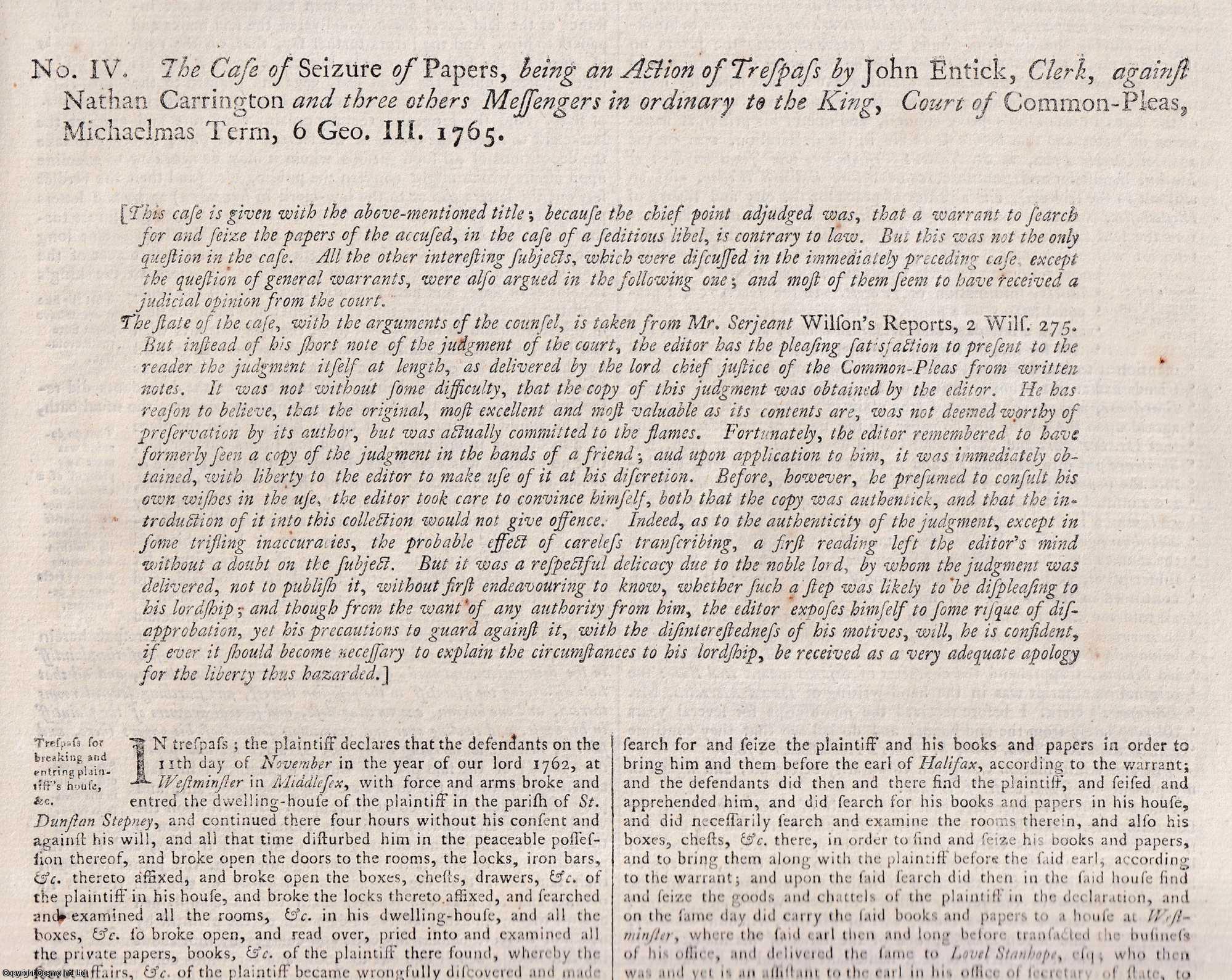This is an image of an old legal document from 1765, titled "Number Four: The Case of Seizure of Papers Being an Action of Trespass by John Entick, Clerk, Against Nathan Carrington and Three Others, Messengers and Ordinary to the King, Court of Common Pleas, Michaelmas Term 6 Geo III." The document is densely packed with text, which appears in a format reminiscent of an 18th-century newspaper. The text is predominantly black and printed on aged, grayish paper, which shows some signs of wear and fading in certain areas. There are also visible signs of text bleeding through from the reverse side of the paper. Noteworthy is a small orange blotch on the right side of the paper. The initial paragraph likely serves as an introductory description in italicized text, followed by content that eventually splits into two columns.